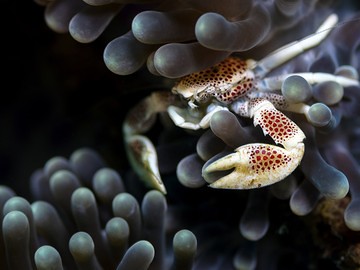The image depicts a small cream-colored crab with reddish-black spots, nestled within a dark, underwater environment. The crab appears to be partially hidden among soft, bristle-like structures that resemble seaweed or some type of flexible plant life, which are gray to black in color. The dark background enhances the contrast, making it initially challenging to distinguish the crab, which has both claws visible and slightly open, as if in a relaxed state. The crab's legs cling onto the surrounding plant material, blending seamlessly with the environment as it rests quietly, its pattern reminiscent of a leopard's spots subtly scattered across its body and claws.